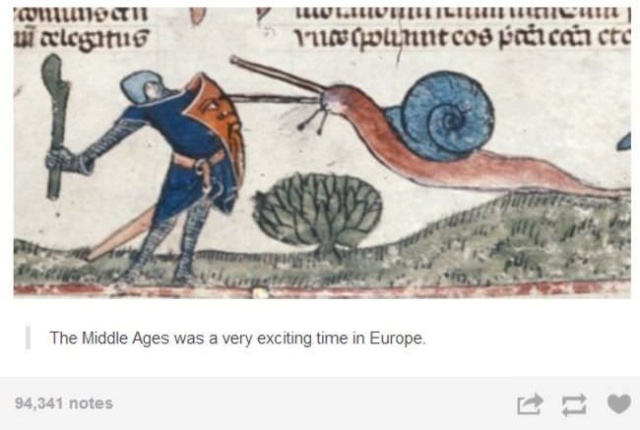The image is a detailed, close-up illustration that appears to be an old piece of medieval artwork, likely originating from a different country. The setting is the Middle Ages, and the scene involves a soldier and a giant snail, both vividly depicted in a variety of colors including dark red, brown, white, gray, light blue, dark blue, orange, and green. The soldier, positioned on the left, is wearing an orange copper breastplate, a blue gown, and a gray helmet. He's wielding a gray club in his right hand and carrying a brown shield over his left shoulder, which features a serious face. On the right side of the image, a large orange-and-gray snail with very long antennae and a blue curly shell approaches the soldier’s shield. The background includes a drawing of a tree and a small hill shading in grayish-green, with grass under the soldier’s feet and a bush in the center. There is text at the top in an unrecognized language, possibly hieroglyphics. Beneath the image, a caption reads, "The Middle Ages was a very exciting time in Europe," followed by a social media bar displaying "94,341 notes" and icons for interactions.